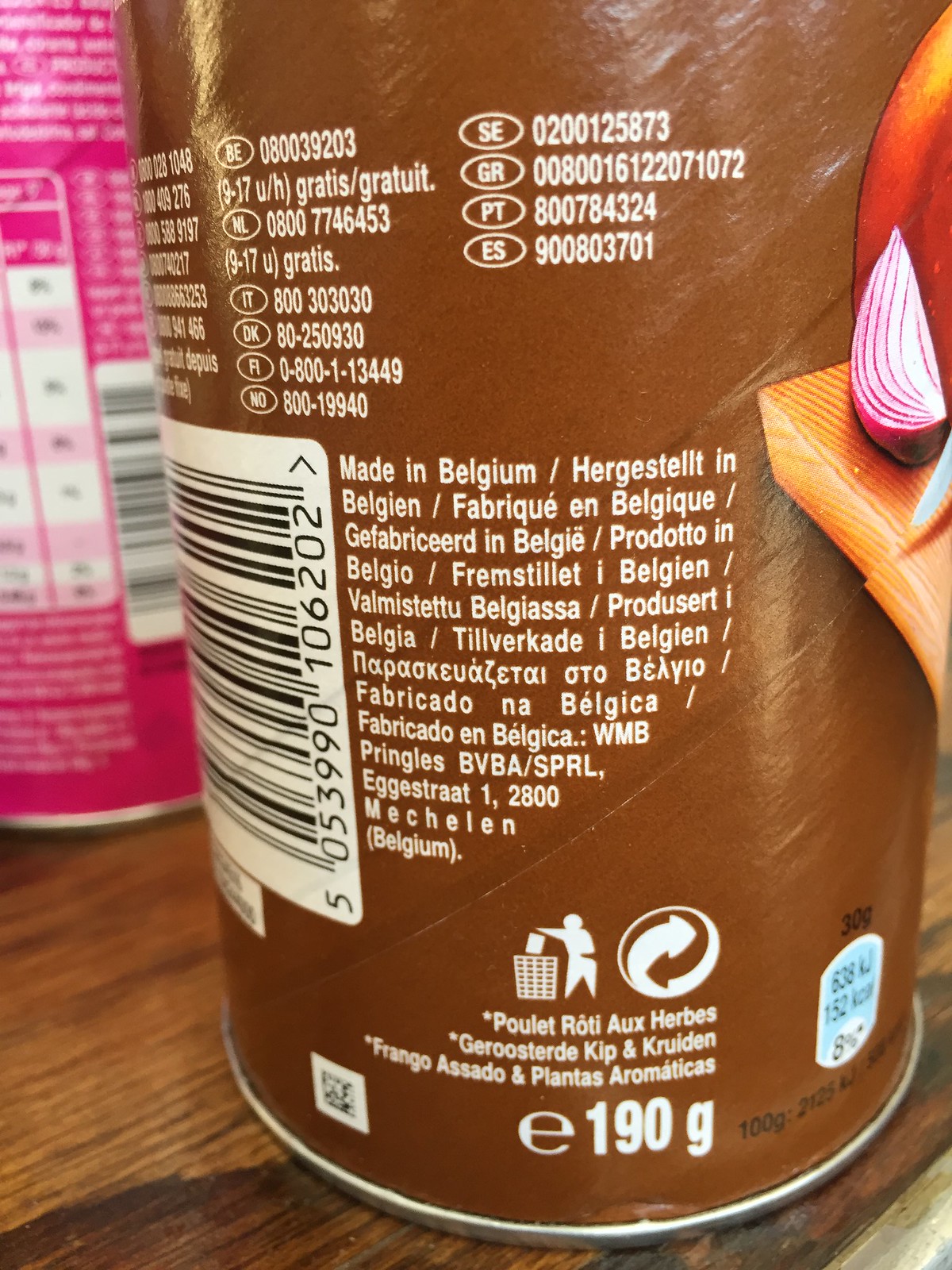The image depicts a detailed view of a brown cardboard container with a metal bottom, positioned on a wooden tabletop. The container's back is filled with white text primarily in Dutch, including the phrase "Made in Belgium" and instructions in multiple languages, likely indicating the product is recyclable. Prominently displayed is a white rectangle housing a barcode and serial number, with "190 grams" labeled near an icon showing a person discarding waste. In the background, a blurred purple container is visible. To the right of the brown container, a cutting board with a knife and a partially chopped red onion slice is seen, adding context to the setting.